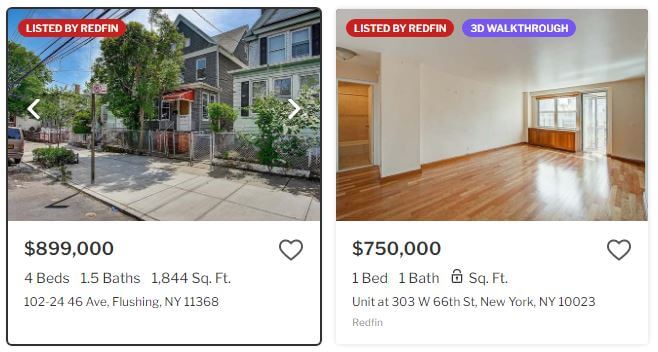The image consists of two side-by-side squares against a white background, each representing a home listing for sale with differing details.

**Left Square:**
- **Image Description:** At the top, a wide-angle photograph captures an urban neighborhood featuring New England-style, two-story homes with white picket fences. The foreground highlights a spacious cement sidewalk and a broad roadway.
- **Redfin Tag:** Located in the top left corner, a prominent red button states "Listed by Redfin" in white text. Adjacent to this are left and right white arrows for navigating through additional images.
- **Listing Details:** The bottom half showcases the listing information. Bold black text displays the price at $899,000, followed by the details underneath: "4 beds, 1.5 baths, 1,844 sq ft" and the address "102-24-46AB Flushing, New York 11368." A small gray heart icon is situated in the upper right corner of this section.

**Right Square:**
- **Image Description:** The top image highlights an interior view featuring polished wooden floors, high ceilings, white walls, and distant windows, suggesting recent renovations.
- **Redfin Tag and Walkthrough Option:** The top left corner also includes a red button marked "Listed by Redfin" in white text. Next to it, a purple button offers a "3D Walkthrough" option.
- **Listing Details:** The bottom portion presents this home’s features on a white background, displaying a price of $750,000 and listing it as "1 bed, 1 bath." The square footage is not specified but noted by a placeholder ("a lock that says square feet"). The given address is "Unit 303, 66th Street, New York, NY 10023," and it’s indicated as listed by Redfin. This section also includes a gray heart icon in the upper right corner.

Both sections include detailed information and functionality to explore further images and interactive options, encapsulating the comprehensive details vital for a home listing.